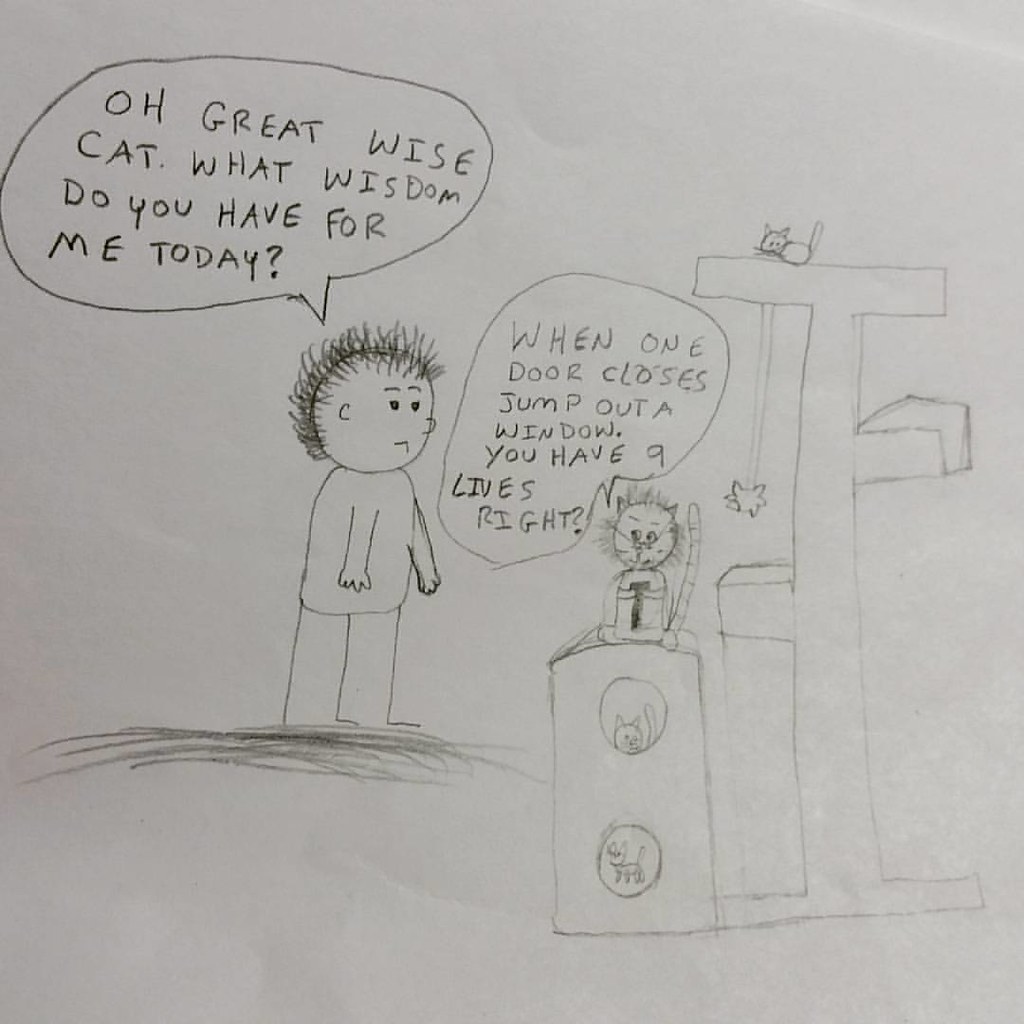This whimsical, pencil-drawn comic on plain white paper appears to be the creative work of a child, evident from the handwriting and sketch style. In the scene, a boy on the left addresses a wise, smiling cat perched atop a cat tree, saying, "Oh great, wise cat, what wisdom do you have for me today?" The cat, positioned above its cat house, replies with a clever piece of advice: “When one door closes, jump out a window. You have nine lives, right?” The cat's expression is cheerful, contrasting with the boy's almost emotionless face. On the right side of the image, another cat playfully drops an object from the top of the cat tree, adding to the comic's charm and humor.